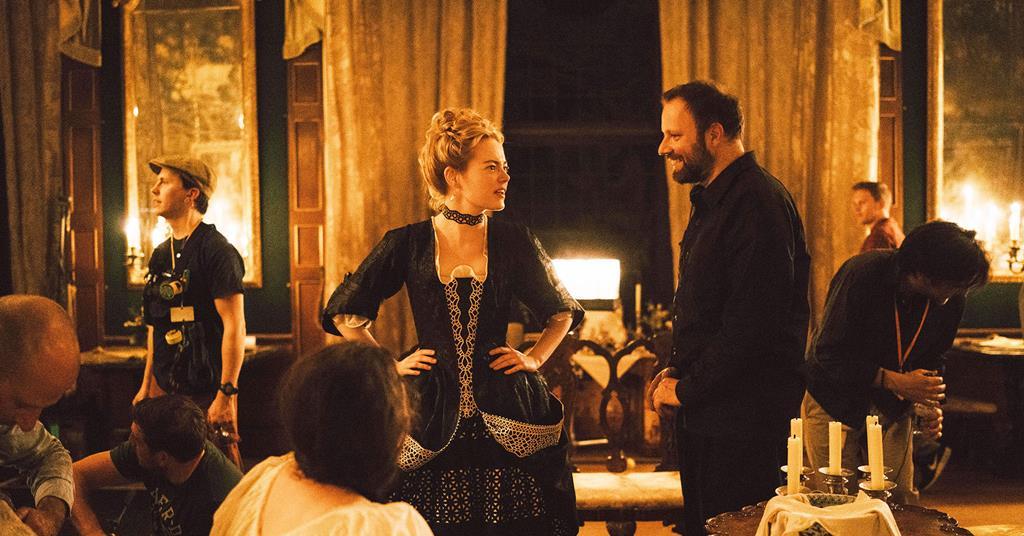The image appears to depict a possible movie set captured in an artistic black, white, and gold opaque tint. Central to the scene is a woman with short blonde hair styled into a bow at the top of her head. She stands confidently with her hand on her hip, adorned in a black dress with a tight, string-pulled bodice, layered over a low-cut blouse and a jacket. A necklace graces her neck. She faces a man in a black suit with a beard, his hands casually in his pockets.

In the background to the right, a young man wearing a cap and a camera slung around his neck looks upwards, possibly at the scene unfolding. To the left, another woman gazes towards the central figures, and a man in a blue shirt looks downwards. Various people, likely workers, populate the background, hinting at the bustling atmosphere of a film set.

The scene is set against luxurious long gold drapes hanging in front of a window, with a large, nearly floor-to-ceiling picture framed in gold visible in the upper right corner. A table in the bottom right holds a three-candled lamp, a bowl, and additional items, adding to the ornate décor. Through the curtains, a door is partially visible, completing the lavish and detailed setting.